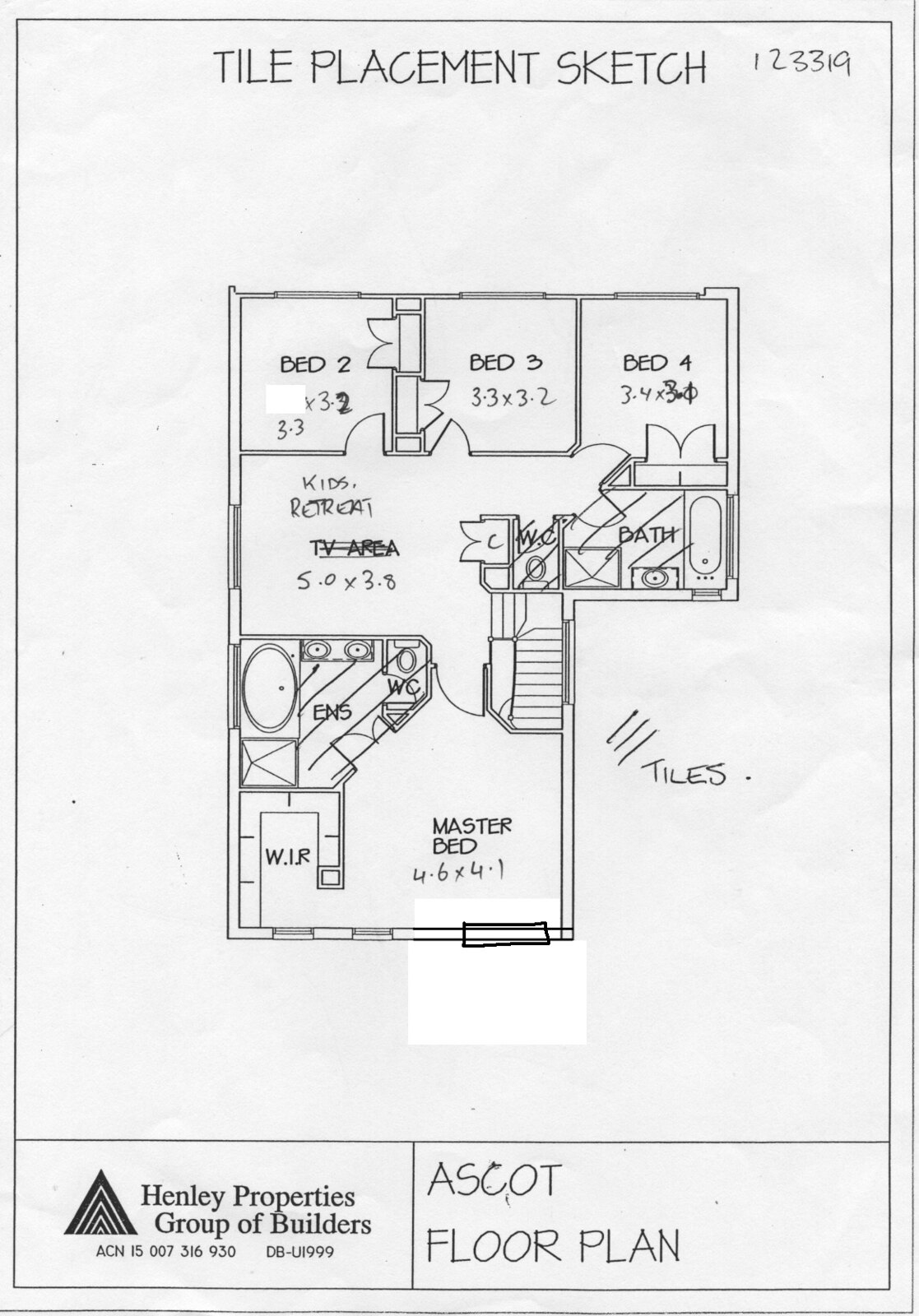This black-and-white image is a detailed floor plan titled "Tile Placement Sketch," prominently displayed at the top. The plan features numeric codes including 1, 2, 3, 3, 1, and 9. The layout is simple and straightforward, beginning with labels for "Bed 2," "Bed 3," and "Bed 4" at the top section. Directly below these bedrooms is an area marked as "Kids Retreat," adjacent to another space that initially says "TB area" but appears to be scratched off. To the right of these zones is a labeled "Bath" area and an adjoining "WC" - Water Closet. Notably, another "WC" area is also indicated, suggesting the presence of two bathroom spaces within the plan. The lower right section of the layout identifies the "Master Bed." Scattered around the plan are stray pen marks, including the word "Tiles." At the bottom-center of the image, it's identified that this floor plan is by "Henley Properties Group of Builders," accompanied by a triangle icon. On the opposite side at the bottom, it reads "Ascot Floor Plan." Additionally, beneath the Henley Properties attribution, a string of numbers and letters is visible, likely denoting a specific project or version code.